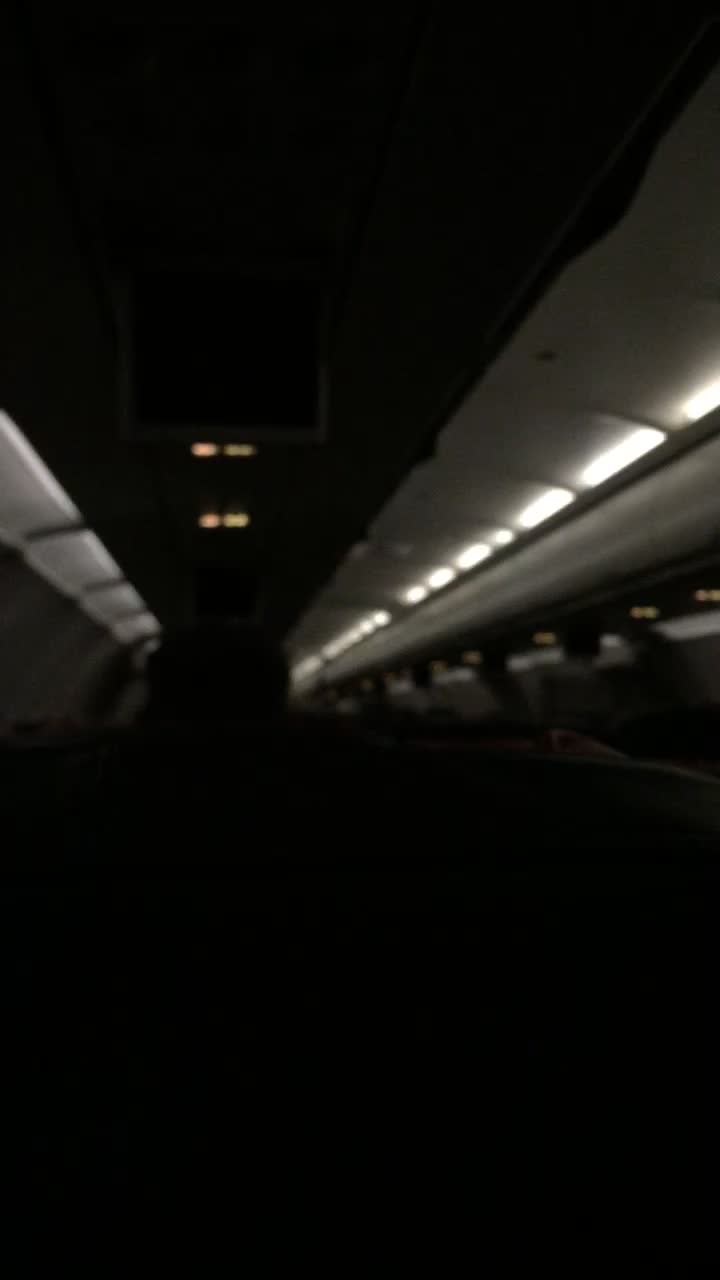A moody, nighttime photograph captures the mystique of a dark tunnel. The inky blackness of the scene is pierced by two rows of bright, white LED lights running along the lower edges of the tunnel, creating a visually striking pathway that seemingly recedes into the distance. Additionally, two small lights peak from the upper part of the tunnel, providing minimal illumination and adding to the overall depth of the image. The stark contrast between the piercing white lights and the enveloping darkness lends an otherworldly ambiance to the photo, highlighting the symmetry and leading lines that guide the viewer’s eye through the tunnel's shadowy expanse.